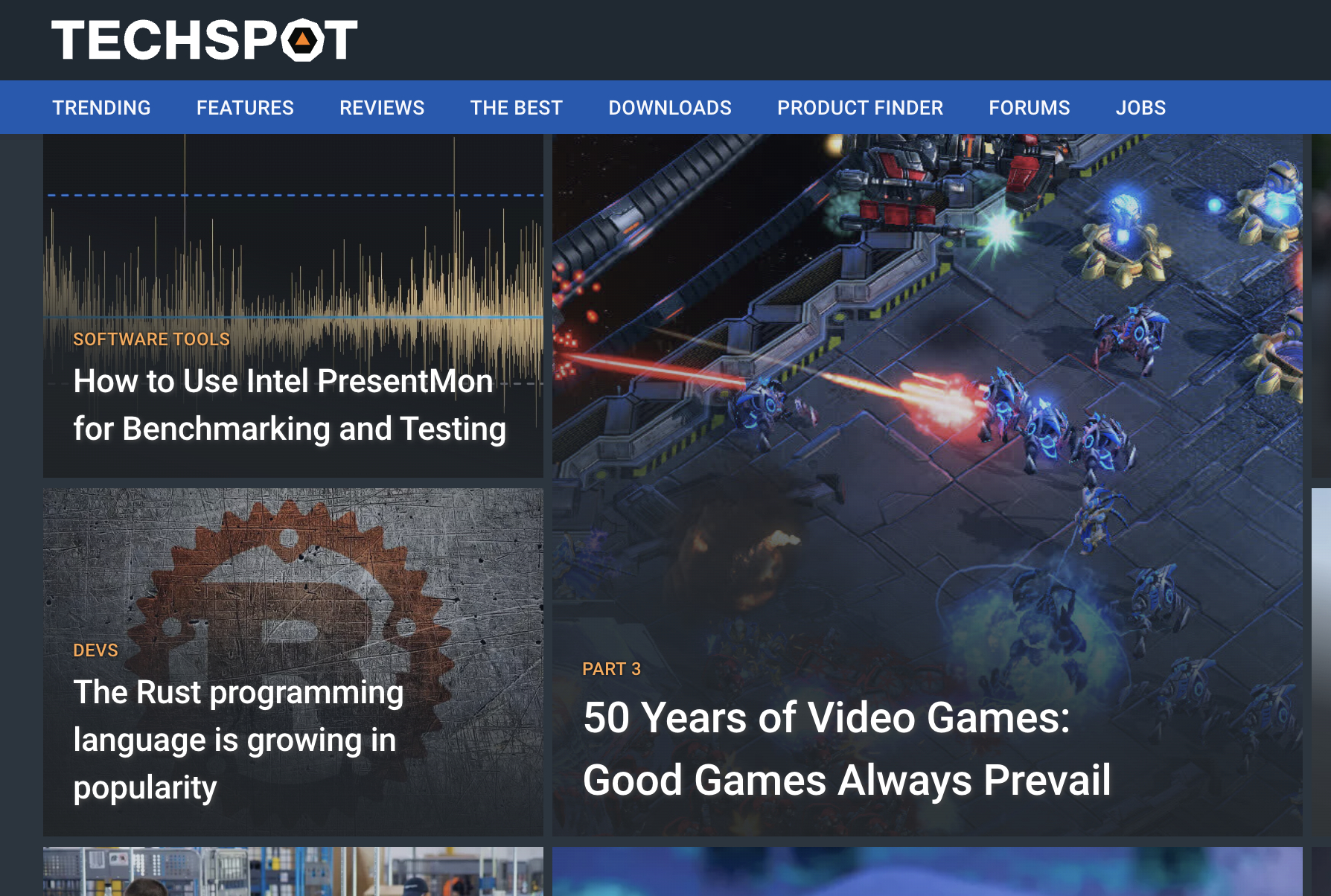In this image against a sleek black background, the top features "Tech Spot" in bold white text, accompanied by a black square embedded within the text and marked with a small red triangle. Below this heading, a prominent blue navigation bar runs across the width of the image, categorically listing "Trending," "Features," "Reviews," "The Best," "Downloads," "Product Finder," "Forums," and "Jobs." 

Underneath, a highlighted section introduces a headline: "How to Use Intel Present Mon for Benchmarking and Testing," labelling it under "Software Tools" with soundwave-like lines that accentuate the technical theme. 

Further down, an eye-catching red circle containing a stylized 'B' marks another segment titled "Devs." This section elaborates on "The Rust Programming Language is Growing in Popularity." On the right-hand side of this segment, an image depicts an intense action scene from a video game where characters are engaged in battle, underscored by the caption "Part 3, 50 Years of Video Games, Good Games Always Prevail." 

At the bottom of the image, two partially visible photos discreetly hint at additional content, teasing the viewer with their incomplete display.